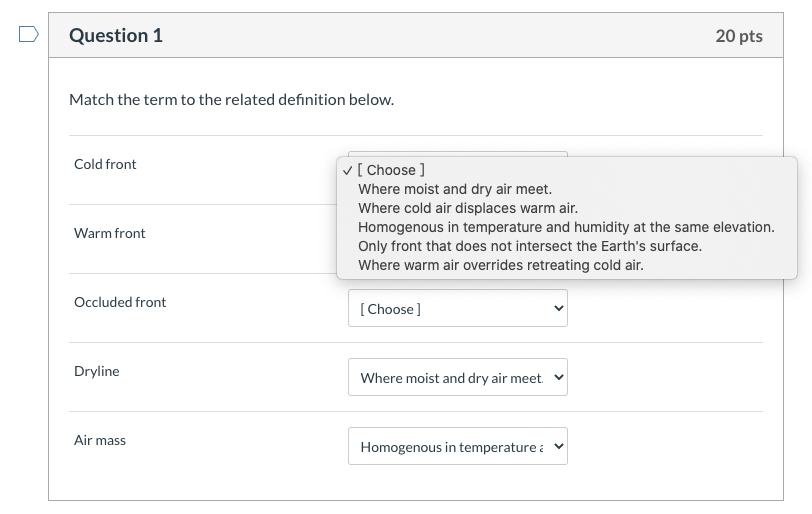A screenshot of an online test or app-based quiz interface is displayed, showing "Question 1" worth 20 points. The task involves matching meteorological terms to their correct definitions using drop-down menus. The question prompt reads, "Match the term to the related definition below."

The first term listed is "cold front," with the options provided in an expanded view:
- where moist and dry air meet
- where cold air displaces warm air
- homogeneous in temperature and humidity at the same elevation
- only front that does not intersect the earth's surface
- where warm air overrides retreating cold air

Other terms such as "warm front," "occluded front," "dry line," and "air mass" follow. However, the drop-down menu for "warm front" is obscured by the expanded "cold front" options. For "dry line," the choice "where moist and dry air meet" has already been selected. For "air mass," the choice "homogeneous in temperature" has been selected. The design of the interface is stark and functional, featuring black and white text with a gray highlight at the top indicating the question number and point value. No additional colors or images adorn the layout.